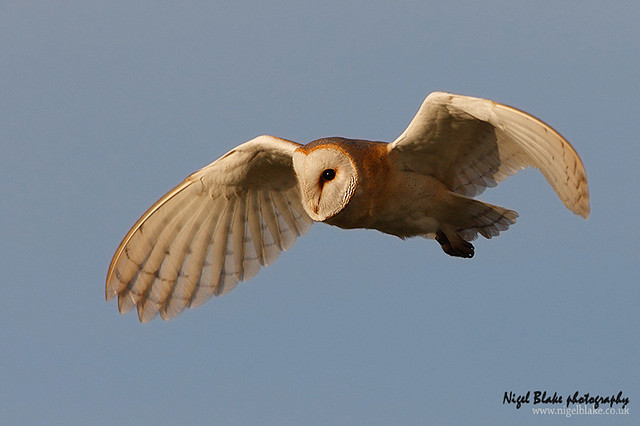The image captures a majestic owl, likely a barn or snowy owl, in mid-flight against a dark grey-blue background suggestive of an evening or nighttime scene. The owl's powerful wings are outstretched, revealing their predominantly white underside with subtle brown tinges towards the top. The bird's head is a mix of brown and white, with a distinctive white face highlighted by a black eye encircled by an orange-brown hue. The owl's body and tail feathers exhibit a brownish tint with visible line patterns. Located in the bottom right corner, the text "Nigel Blake Photography" is elegantly inscribed in black cursive, with "www.nigelblake.co.uk" printed in white underneath. The photograph appears to be a digital or possibly AI-generated image, capturing the breathtaking scene from the underneath view of the owl, accentuating its graceful flight across the dark backdrop.